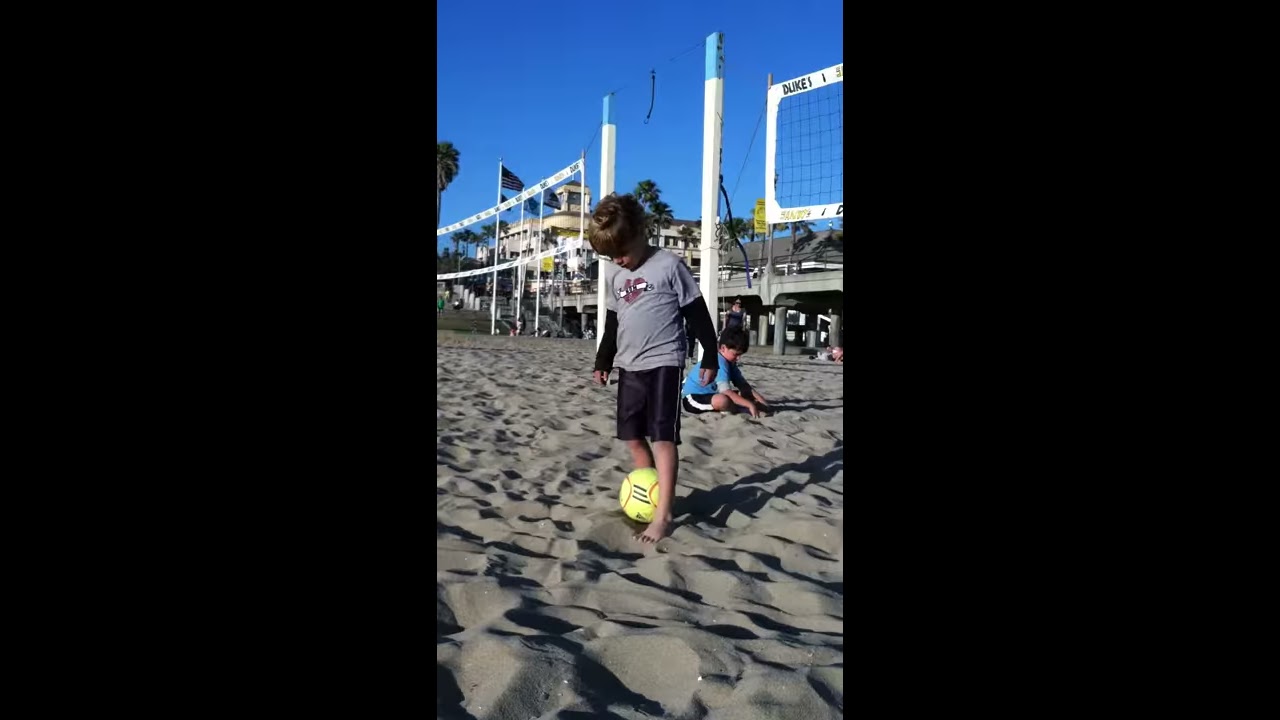In this detailed photograph, a young boy stands barefoot on a sandy beach volleyball court, preparing to kick a mostly yellow soccer ball adorned with white spots and red outlines. The sand underfoot creates an uneven surface of small bumps and troughs. He wears black shorts and a gray short-sleeved shirt layered over long dark sleeves. His thick head of hair and focused downward gaze add to the scene's detail. To his left, another boy in an aqua blue shirt and black shorts with white stripes sits on the sand near a white support beam of a volleyball net, playing with the sand and looking towards the right. The photograph is framed within a horizontal rectangle with a black border on the left and right sides that occupies two-thirds of the picture's width. In the background, there are two volleyball nets supported by white pillars with bluish tops, a distant building with an elevated area possibly resembling a pier, a walking slope to the left of the building, and a palm tree to the left. The sky overhead is a clear blue, adding to the bright and lively outdoor daytime beach setting.